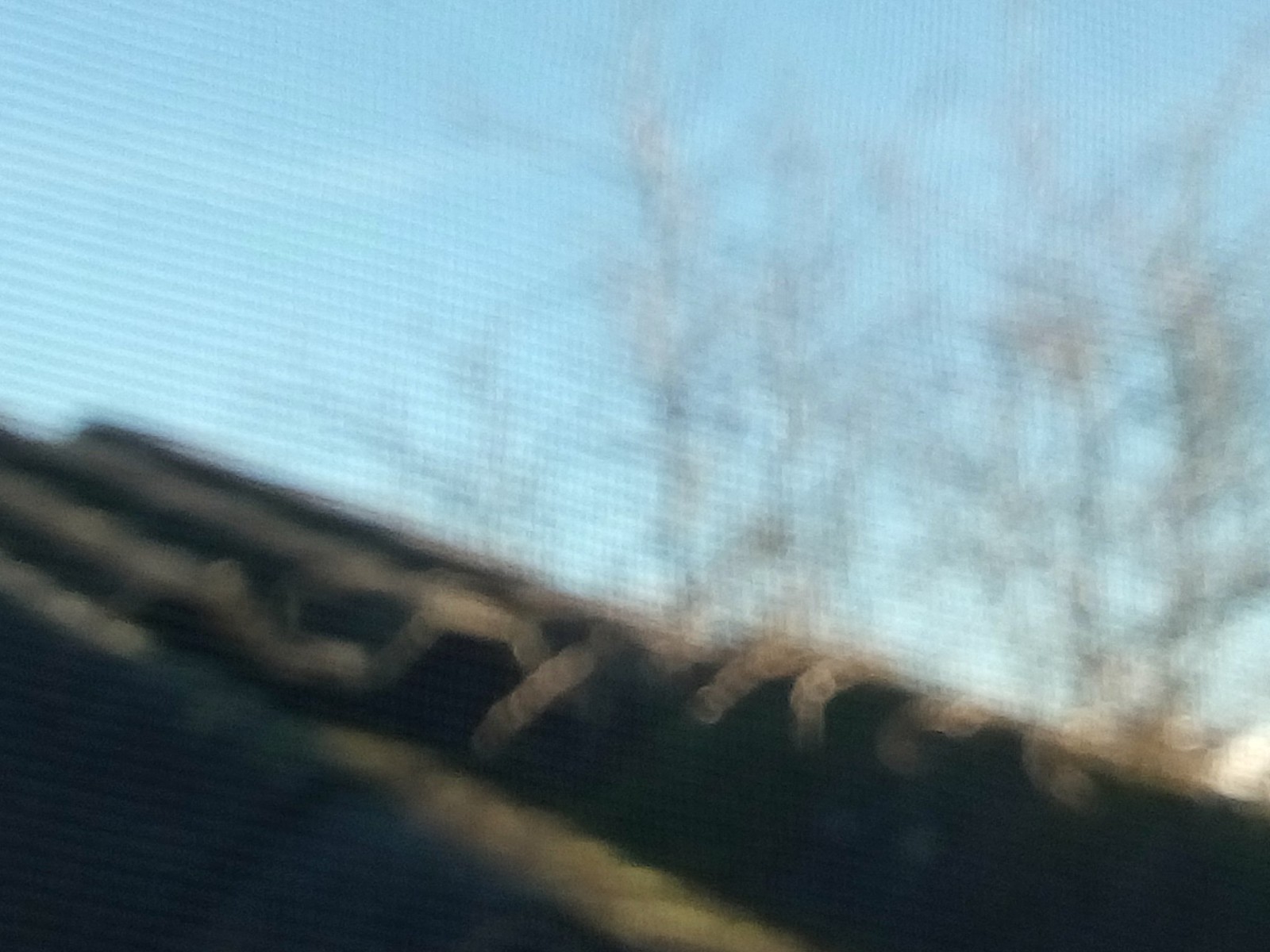This is an extremely blurry and zoomed-in photograph taken outdoors, seemingly through a screen that adds a mesh-like filter over the entire image. The focal point appears to be a structure or possibly stacked logs or pipes, extending from the bottom right to the center left of the picture. Behind this, one can faintly make out tall, leafless trees, suggesting it might be winter. The sky is a clear, baby blue with a few scattered white clouds visible at the top. The overall poor quality and blurriness of the photo, combined with the screen overlay and likely camera movement, make it difficult to discern precise details. The photographer might have been experimenting with different techniques, though with less successful results.